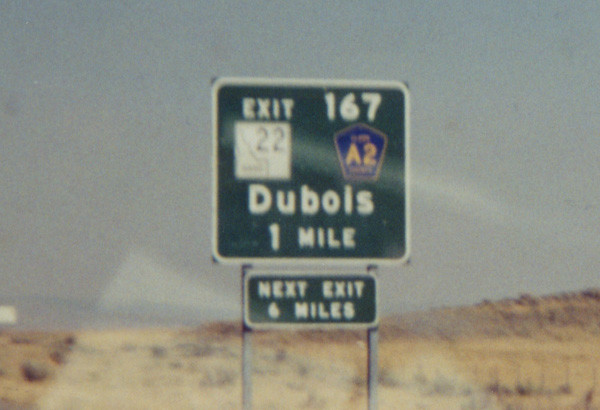The image depicts a low-resolution, somewhat grainy photograph of an interstate road sign situated in a desert area with brown sandy ground and sparse scrubby vegetation. The green sign with a white border prominently displays "Exit 167" alongside a small white rectangle labeled "22." Below this is a highway symbol in blue with yellow letters "A2," and beneath that, it reads "Dubois 1 mile" in white letters. Another rectangular sign below it, green with a white border, states "Next exit 6 miles." The signs are mounted on two gray metal poles. The background includes a brown hill with minimal vegetation and rocks in the lower-left corner. The sky is a grayish-blue without any visible clouds. There is a noticeable reflection, likely from a car windshield, casting a white line across the upper sign and contributing to the image's overall blur.